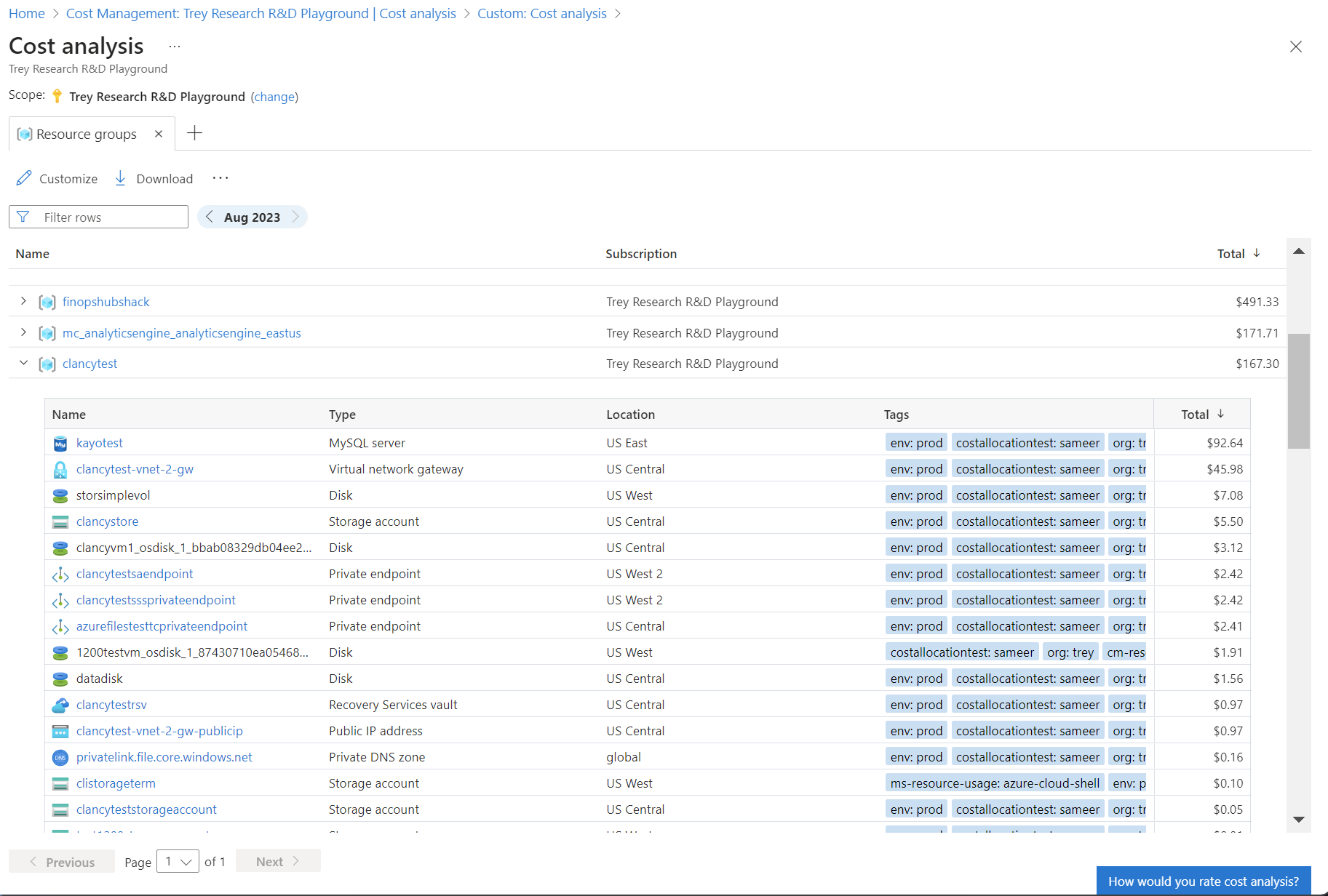An extensive spreadsheet, titled "Cost Analysis, Trey Research R&D Playground," fills the screen. In the upper left corner, the title is prominently displayed. On the upper right corner, there's an option to close the document, marked by an "X." Below the title, "Scope, Trey Research R&D Playground" is mentioned, with a blue parenthetical note, "Change."

A tab labeled “Resource Group” organizes the data further, and beneath it are options to "Customize and Download" followed by ellipses, indicating additional settings or features. Another section offers a "Filter Rows" option and a button for navigation. Navigational arrows (left and right) flank the date "Aug 2023," with the arrows styled in a light blue hue, distinguishing them against the primarily white or light gray background.

The upper left corner hosts textual details, "FinopshubShack, McAnalysisEngine, underline, AnalixEngine, underline, Eastus," indicating specific analysis tools or segments. Below this section lies another test entry named "Clancy test."

The main body of the spreadsheet is compartmentalized into columns labeled “Name, Type, Location, Tags, Total.” The first entry reads: "KO Test," under the "Name" column, described as a "MySQL Server" in the "Type" column, located in "US East." The "Tags" column includes detailed metadata: "ENV: Product, Coast: All, Location: Test, ER, Org: TR." The total cost for this entry is listed as $29.64.